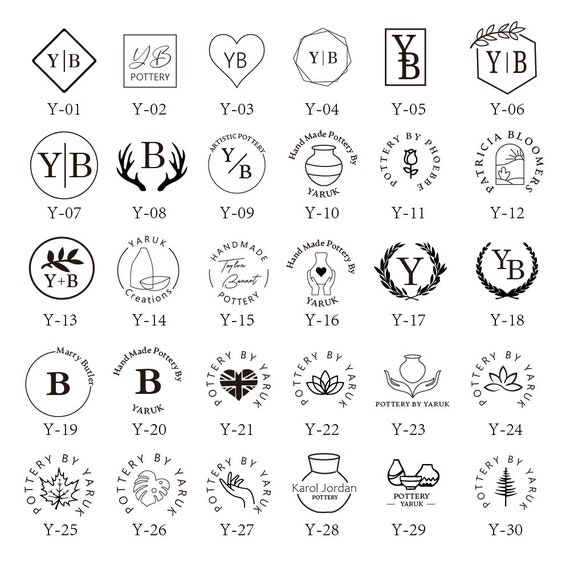The image is a black and white, square-shaped grid depicting five rows of labeled logos used by a company or individual possibly named "Pottery by Yaruk." Each logo features different shapes such as diamonds, squares, hearts, octagons, rectangles, and hexagons, and they all contain the letters "Y" or "YB" in various stylized forms. The logos are organized sequentially from top left to bottom right, beginning with Y-01 and ending with Y-30. Each logo is accompanied by an identifier label beneath it, starting from Y-01, moving rightward to Y-06 in the first row, Y-07 to Y-12 in the second row, and continuing this pattern till Y-30 in the bottom right corner. Notably, some logos include design variations such as lines or additional elements like an olive branch, enhancing their visual complexity while maintaining the Y or YB theme.